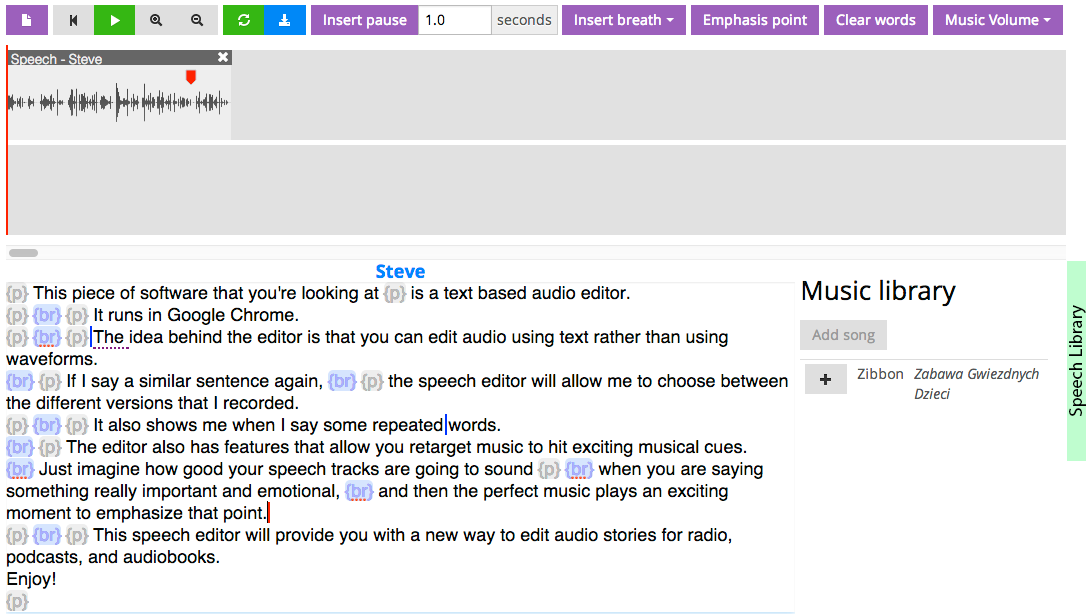A screenshot of a text-based audio editor running in Google Chrome is shown. At the top, there's a menu bar featuring various icons including a page, start over, play, zoom in, zoom out, refresh, download, insert, pause, and other functions related to audio editing. The main interface is divided into two main sections. The top section displays a single waveform labeled "Speech - Steve," indicating audio content. A red arrow, presumed to be the playhead, is positioned approximately 80% along the timeline. The lower section is filled with text, seemingly a transcription of the audio, with numerous annotations such as "insert breath," "emphasis point," and "clear words," similar to HTML tags. 

The text explains the purpose of the editor, noting that it allows users to edit audio using text commands rather than traditional waveform manipulation. It highlights features such as the ability to choose between different recorded versions of a sentence and retargeting music to match speech. The editor aims to enhance audio storytelling for radio, podcasts, and audiobooks by allowing precise control over speech and musical cues.

On the right side of the interface, there are two sections: the "Music Library," which includes an add song function marked by a plus button, and a "Speech Library," indicated by a green vertical line.